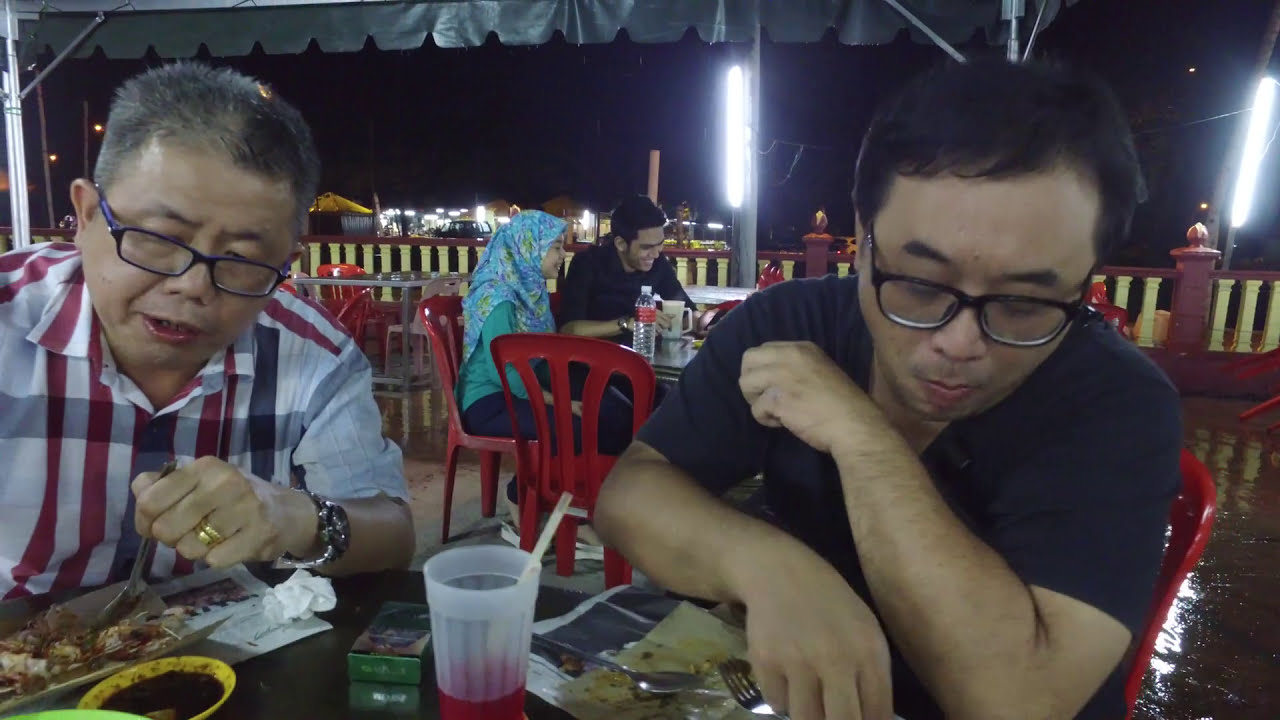In this nighttime outdoor restaurant setting, two Asian men, possibly a father and son, are the primary focus of the image. They are seated at a round table under a canopy, enjoying what appears to be takeout food served in paper containers, complete with forks and a dipping sauce. Both wear glasses and have short hair; the older man on the left sports black-rimmed glasses and a white short-sleeved collared shirt with red and blue vertical and horizontal stripes. He also has a silver watch and a gold wedding ring. The younger man to his right, wearing a blue short-sleeved shirt, has thicker black-rimmed glasses and similar short black hair. Behind them, a couple can be seen at another round table with red plastic chairs. The woman is adorned in a blue headdress, paired with a long-sleeved green shirt and blue pants, while the man beside her laughs in a blue shirt. The seating area is illuminated by lights on the posts of the canopy, giving a cozy, bustling ambiance to the nighttime dining experience.